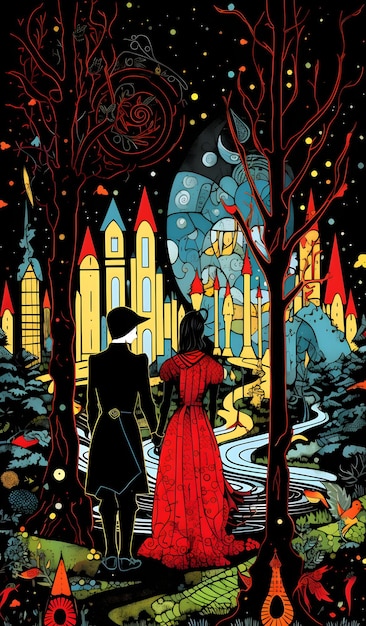This is a detailed illustration featuring a distinctive blend of dark and vibrant colors, reminiscent of stained glass. The focal point is a couple walking through what appears to be a fantastical park. The woman is clad in a long red gown with black sleeves, her black hair flowing behind her. She is holding hands with a man dressed in a long black uniform coat and a black hat, giving off an air of mystery and strength. Both are viewed from the back.

The background is predominantly black, serving as the canvas for an array of colors that bring the scene to life. Tall black trees outlined in red frame the couple, while the sky above is a deep, void-like black, scattered with sparkling dots in vibrant hues of orange, blue, yellow, and green, mimicking planets and stars.

In the distance, the horizon is adorned with tall yellow buildings topped with pointy red and blue roofs, evoking the look of a fantastical castle or ancient towers. Swirling blue pathways, possibly roads or rivers, wind through this whimsical landscape. The foreground includes trees, plants, and other natural elements, contributing to the scene’s enchanting, otherworldly aesthetic.